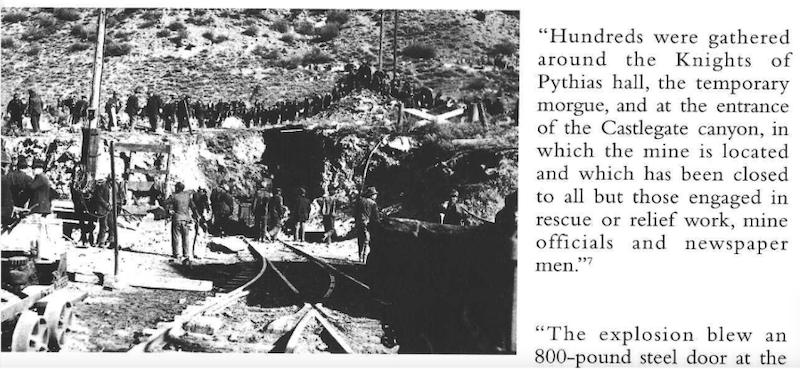This black-and-white photograph, featured alongside a printed newspaper article, captures a poignant moment at a mine site. The vintage-style image is set in landscape orientation with the photograph occupying two-thirds of the space on the left, and the article text in a single column on the right. In the dimly lit photograph, numerous workers can be seen gathered around intersecting sets of mine car tracks that lead into a dark tunnel, suggesting the mine entrance. Above the tunnel and beside the tracks, more workers are lined up, emphasizing the gravity of the situation. The accompanying article reads, "Hundreds were gathered around the Knights of Pythias Hall, the temporary morgue, and at the entrance of Castle Gate Canyon, in which the mine is located and which has been closed to all but those engaged in rescue or relief work, mine officials, and newspapermen." The text further mentions, "The explosion blew an 800-pound steel door," though it is partially cut off. This detailed image and article reflect the aftermath of a tragic mining explosion and the collective efforts of rescue and relief personnel.